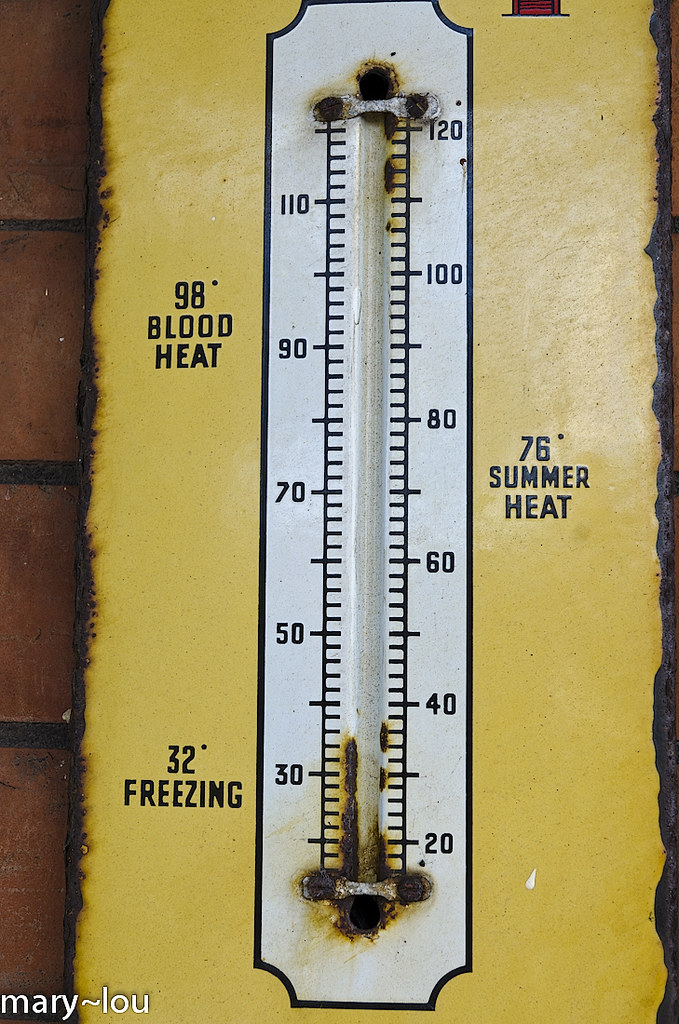This image captures a vintage thermometer set against a backdrop of a rich, golden-yellow material, which appears to be either metal or cardboard. The thermometer itself is encased in glass, showing signs of aging with noticeable rust and black discoloration at its base. The temperature scale is detailed with numbers clearly marked on both sides of the thermometer: on the left, it lists 110, 90, 70, 50, and 30 degrees, while the right side features 100, 80, 60, 40, and 20 degrees.

Distinctive markers indicate specific temperatures: at 98 degrees, the label reads “blood heat,” at 76 degrees, it denotes “summer heat,” and at the bottom of the scale, 32 degrees is marked with the word “freezing.” 

The thermometer is positioned in front of a red brick surface, which adds a rustic charm to the overall image. At the very bottom, the name “Mary Lou” is inscribed in a script font, adding a personal touch to this nostalgic scene.